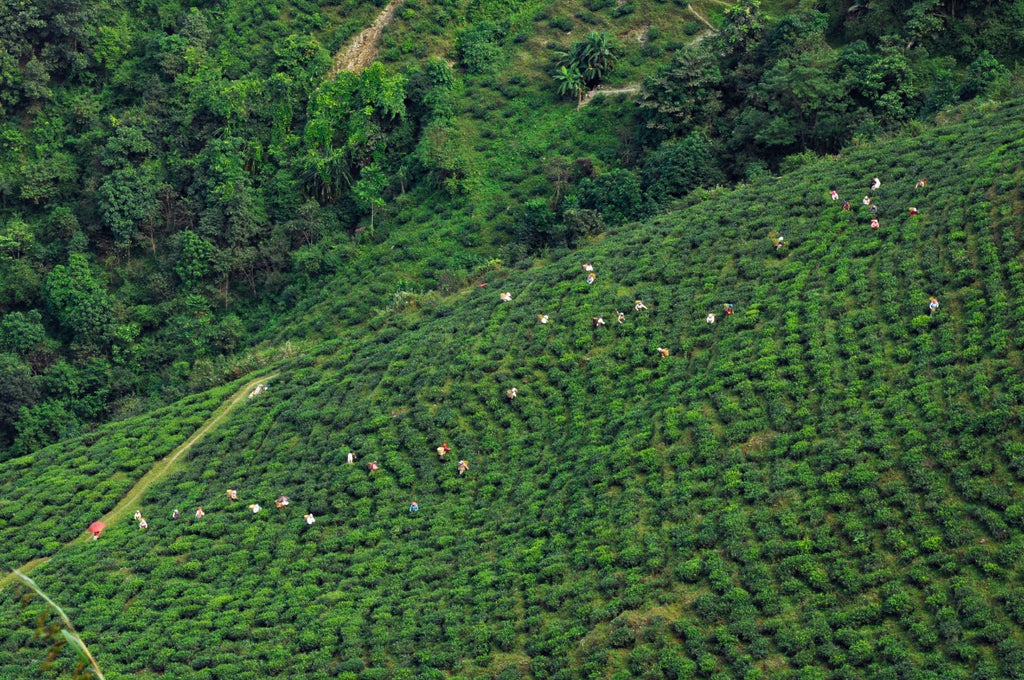In this somewhat aerial, zoomed-out photograph, we see a vast, vibrant green field with high levels of lush vegetation. The field appears to be cultivated, likely a crop field with rows of round bushy plants that resemble cabbage or lettuce. Tiny white specks, presumably farmers, are scattered throughout the greenery, working diligently. The farmers, bending over with something on their backs, are arranged in a line stretching diagonally from the bottom left corner to the top right corner, suggesting they are harvesting crops. In the background, there's a dense, wild green forest contrasting with the more orderly cultivated field. A distinct, cleared path cuts vertically near the bottom left corner of the image, acting as a boundary or walking passageway through the field. Amidst the greenery, one can also spot a person holding a red umbrella near this path. It is a bright daytime scene, shot from above, focusing downward onto the field, highlighting the farmers' efforts amidst nature's abundant greenery.